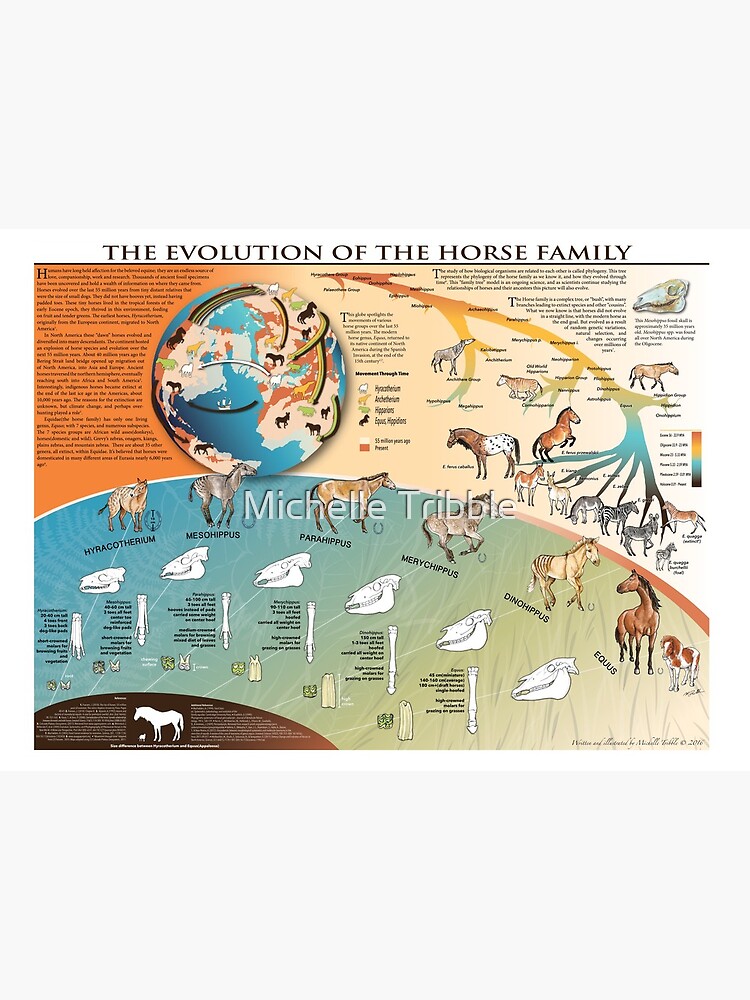This highly detailed educational poster titled "The Evolution of the Horse Family" provides a comprehensive visual history of the horse lineage through colorful, illustrative elements. The upper half of the chart predominantly features an orange-to-white gradient background with various paragraphs of text that delves into the evolutionary journey of equines, though the text is not easily readable. Prominently, a cartoon illustration of the globe occupies the upper left corner, highlighting key migration paths of ancient horse ancestors across different continents.

To the upper right, a detailed family tree maps out the progression from prehistoric horses to the modern horse. This tree branches out from various root animals, showcasing an array of early horse species that culminate at the modern Equus positioned towards the page's right edge. Key landmarks along this evolutionary path are underscored through their Latin names, and precise illustrations of their skulls and leg bones placed alongside their respective full-body depictions.

A distinct watermark in white shaded lettering at the center reads "Michelle Tribble," likely indicating the chart's creator. The lower portion of the poster is adorned with an arc that transitions from blue and gold gradient tones to dark browns and reds, encapsulating the detailed skulls, leg bones, and scientific illustrations of seven distinct horse species. Each species is neatly labeled with its Latin name, enhancing the educational value of the chart. The vivid palette used throughout—from deep orange and blue to green and tan—adds to the visual appeal, making the complex evolutionary history more engaging and accessible.